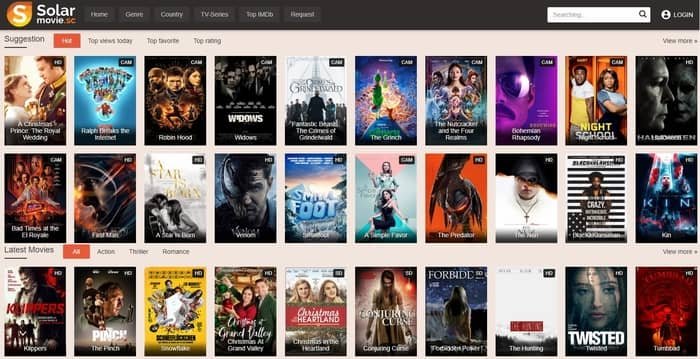A screenshot from a web page displaying the SolarMovie streaming platform. At the top of the page, there is a stylized "S" logo within a teardrop-shaped icon featuring a gradient of red, orange, and yellow hues. Below the logo, a navigation bar includes options such as "Home," "Center," "Genre," "Country," "TV Series," "IMCO," and "Request." The main display area of the page features three full rows of movie thumbnails, each row containing ten movie posters—30 in total.

In the top row, the movie titles are: "A Christmas Prince: The Royal Wedding," "Ralph Breaks the Internet," "Robin Hood," "Widows," "The Gardener," "The Grinch," "The Nutcracker and the Four Realms," "Night School," and "Halloween." The titles in the remaining two rows are not detailed in the description provided. The overall layout is clear and organized, showcasing a variety of film genres available for streaming.